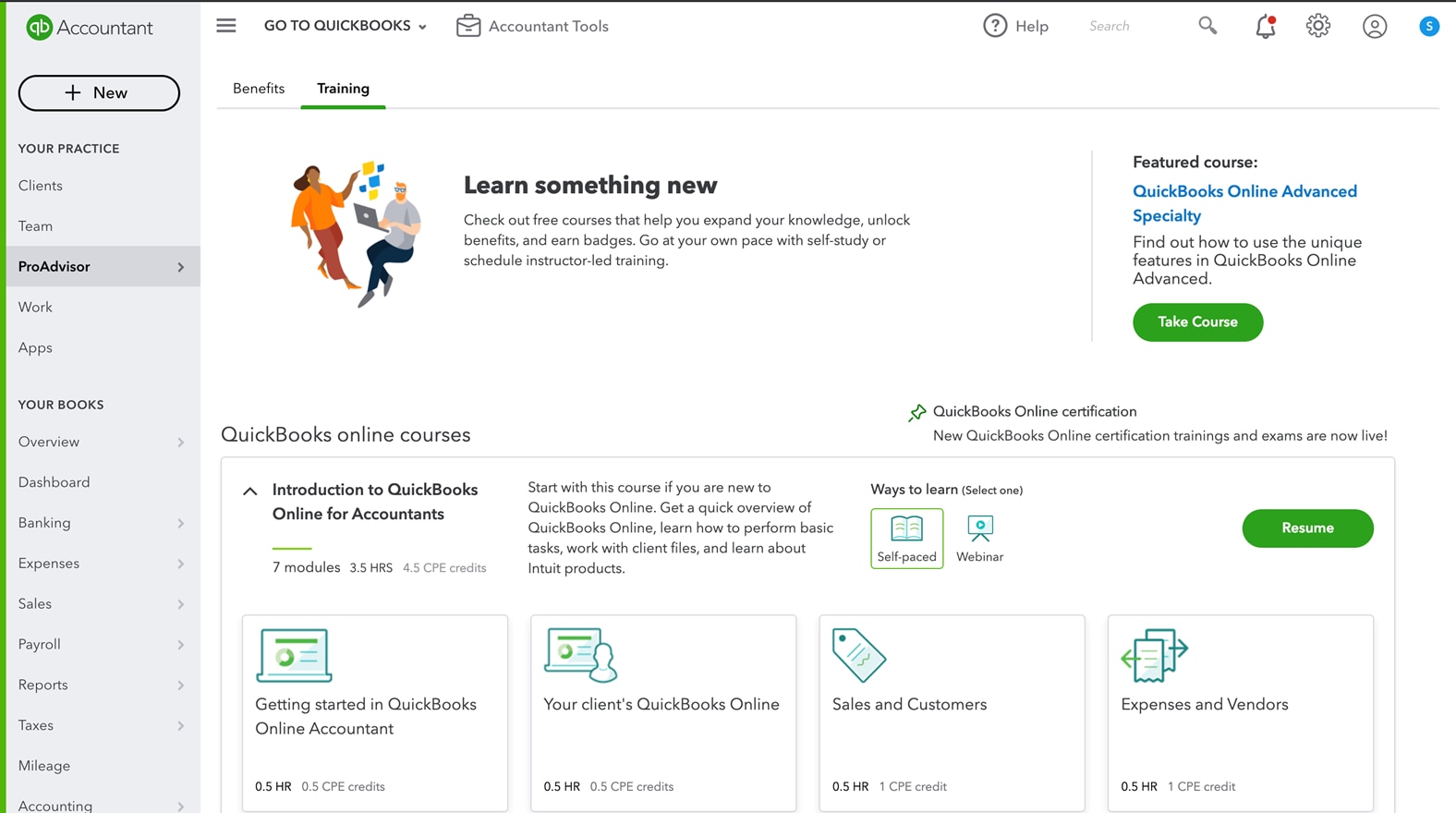The image captures the user interface of QuickBooks accounting software, featuring a comprehensive dashboard designed for accountants. In the top-left corner, the screen displays "QB Accountant" and "New," indicating that this view is tailored for accounting professionals. The left sidebar presents a series of navigation options including "Your Practice," "Clients," "Team," "ProAdvisor," "Work," "Apps," "Your Books," "Overview," "Dashboard," "Banking," "Expenses," "Sales," "Payroll," "Reports," "Taxes," "Mileage," and "Accounting." Many of these categories have expandable sub-menus for further navigation.

On the top-right corner, the interface features quick access buttons such as "Go to QuickBooks" with a dropdown, "Accountant Tools," "Help," "Search," "Notification Icon," "Settings," and a low-profile user icon next to a small "S," the purpose of which is unclear.

The main section of the screen prominently highlights training and certification resources. Under the heading "Benefits or Training," users are encouraged to check out free courses that help expand their knowledge, unlock benefits, and earn badges. The text emphasizes the flexibility of self-paced study or the option to schedule instructor-led training. A colorful illustration accompanies this section, depicting a white male with red hair and a laptop, and an African-American female with long hair, dressed in vibrant clothing, symbolizing the diverse learning community.

To the right, the screen showcases "QuickBooks Online Certification," promoting new training courses and exams. The "Featured Course" spotlight emphasizes "QuickBooks Online Advanced Specialty," inviting users to explore the unique features of QuickBooks Online Advanced through the "Take Course" button.

Lower down, the "QuickBooks Online Courses" section offers an introductory course named "Introduction to QuickBooks Online for Accountants," consisting of seven modules totaling 3.5 hours, and providing 4.5 CPE credits. The course is ideal for new users, covering basic tasks, client file management, and Intuit product knowledge. Learning methods include self-paced options and webinars, with a "Resume" button indicating that the user has already initiated the course. Further detailed modules include:

- "Getting Started in QuickBooks Online Accountant" (30 minutes, 0.5 CPE credits)
- "Your Client's QuickBooks Online" (30 minutes, 0.5 CPE credits)
- "Sales and Customers" (30 minutes, 1 CPE credit)
- "Expenses and Vendors" (30 minutes, 1 CPE credit)

The image effectively portrays the robust training infrastructure within the QuickBooks accounting software ecosystem, designed to support accountants in their professional growth.